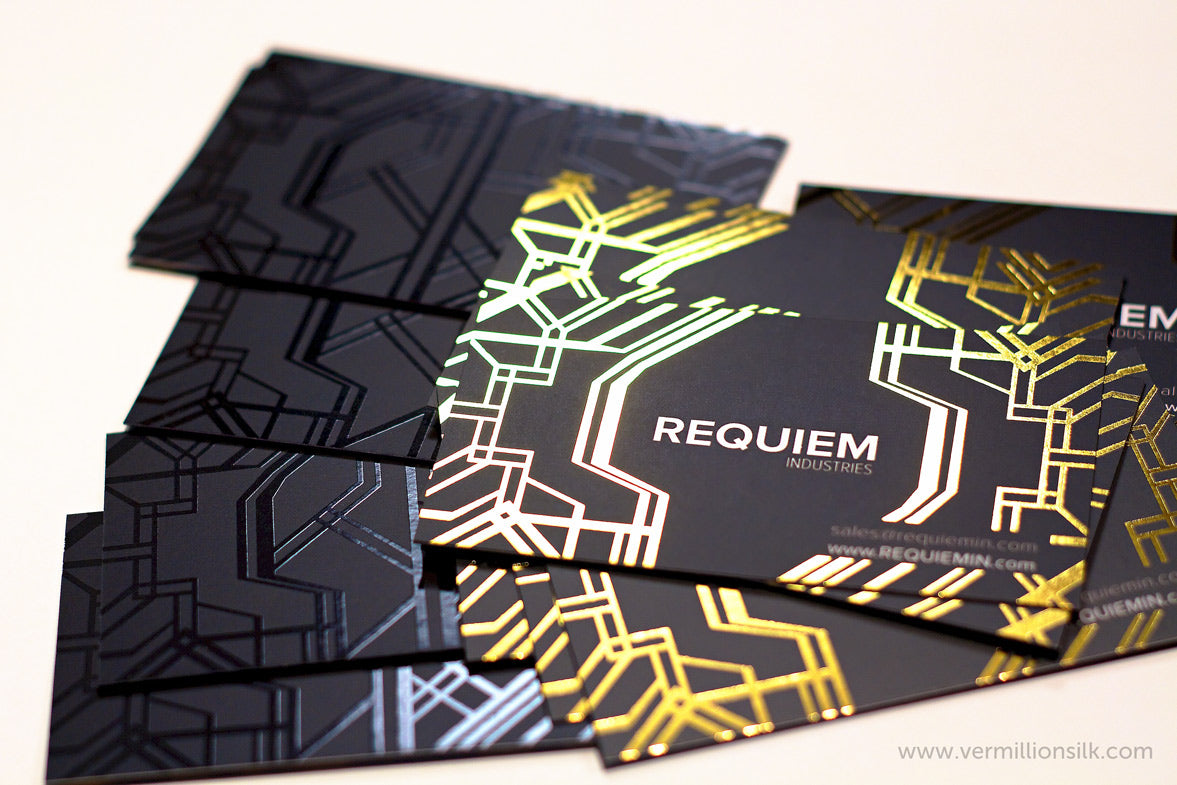The image displays a stack of sophisticated business cards scattered across a light-colored, off-white surface. The majority of the cards visible are black, adorned with intricate geometric patterns. A significant portion of these cards showcase glossy black patterns, while some are embellished with glossy blue designs. The most eye-catching feature belongs to a stack of cards positioned centrally and to the right, which boast vibrant golden-yellow and pale-yellow geometric lines against a black background. Each of these cards prominently displays the words "Requiem Industries" in white text. In the bottom right corner of these golden-patterned cards, the website "www.requiem.com" is clearly visible. To the left, a separate stack of cards hints at a similar geometric design but remains understated with glossy black patterns on a matte black background, devoid of any written information. The arrangement provides a visual contrast, emphasizing the elegance and modernity of the designs.